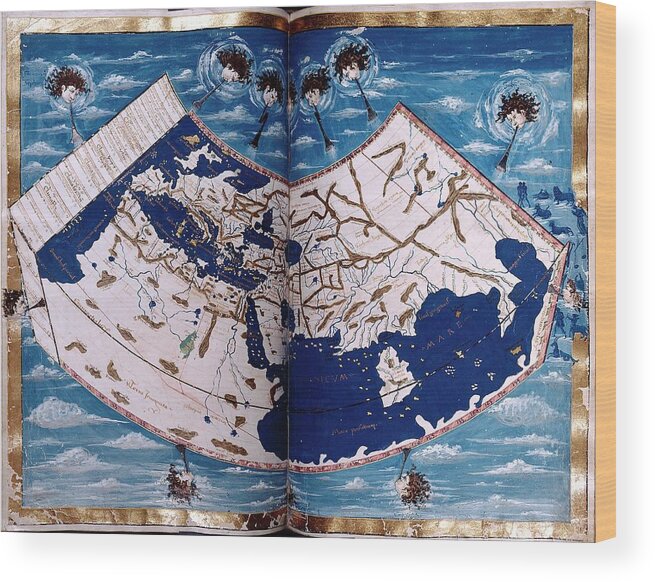This image features an open book with golden matte edges, appearing as a 15th-century map possibly printed on wood or thick pages. The map spans both pages of the book, depicting a detailed cartography showcasing a variety of topographical elements such as white-colored lands accented with brown splotches, likely indicating cities, rivers, lakes, or routes. Blue sections are visible, representing waterways. Surrounding the map are artistic representations of men's heads with dreadlock hairdos blowing pipes, reminiscent of mythological winds. The background of the map adds to its elegance, with a blue hue and intricate designs. The gold accents around the book lend an air of antiquity, enhancing its historical aura.